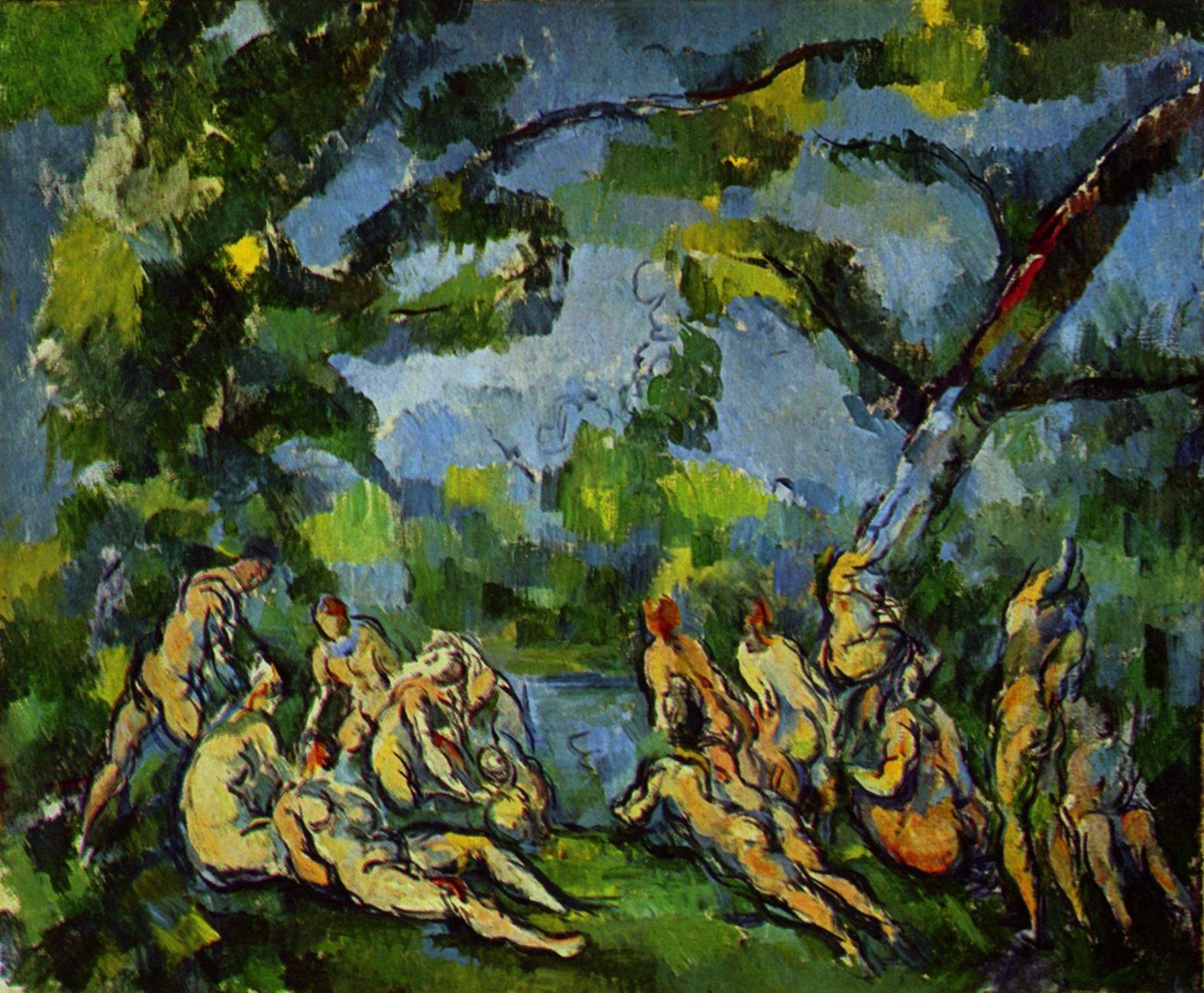The painting depicts a natural, green landscape dominated by several trees and various forms of vegetation. In the background, a serene blue sky transitions into a body of water, possibly a lake or pond, adorned with hints of green vegetation. There's a collective of 13 nude individuals of indeterminate genders scattered across the lush green grass at the painting's forefront. These figures, with hair colors ranging from black to brown to red, are depicted in different states of relaxation—sitting, lying down, or standing. The brushstrokes suggest the work of a notable artist, giving the scene a somewhat indistinct, dreamlike quality. The people are positioned in a way that they're mostly facing away or each other, contributing to the sense of calm and contemplative atmosphere in this subtly lit daytime setting.